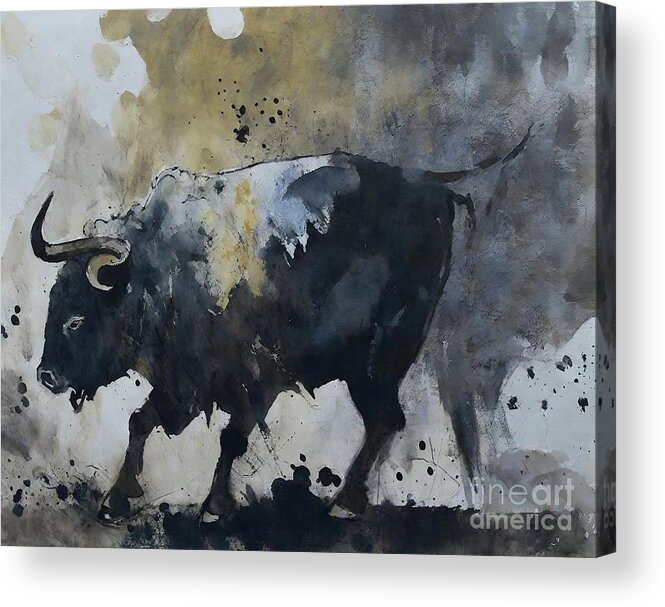This image is a painting, possibly done with watercolors or oils, depicting a dynamic scene of a bull, or perhaps a bison. The animal, primarily black with a distinctive white patch on its upper back, is shown in a powerful stance that suggests it is kicking up dirt from the ground. Its two prominent horns, large nostrils, and black eyes give it a fierce expression as it faces towards the left side of the painting. The background consists of a muted swirl of grays, blacks, mustard yellows, and blues, creating a cloudy, somewhat tumultuous atmosphere. There are splatters of black paint throughout, adding to the sense of motion and energy in the scene. The lower right-hand corner of the image contains a watermark in pale white-gray font reading 'Fine Art America'. The ground beneath the bull blends into the painting's dark tones but is distinct enough to highlight the animal's movement and posture.